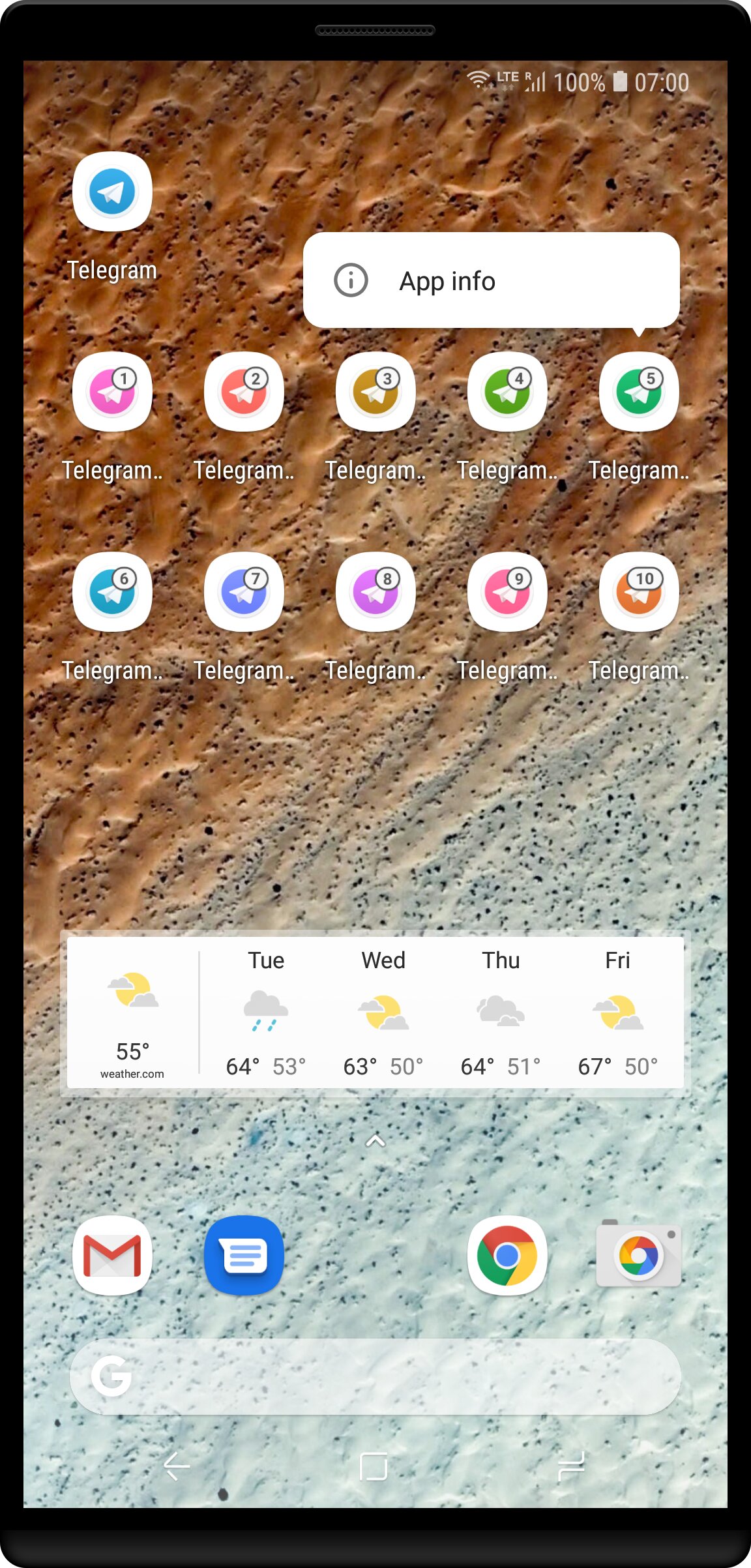The image displays a screenshot from a cell phone featuring a beach-themed background. The top half of the screen is dominated by a sandy texture transitioning into a foamy wave-like appearance towards the bottom, mimicking the shoreline. Observably, the phone's battery is fully charged at 100%, and the time displayed is 7:00.

The home screen showcases multiple instances of the Telegram app icon arranged in a grid. The topmost icon is a standard Telegram icon. Below it, there are various Telegram icons in an array of colors: pink, orange, burnt yellow, green, and a lighter shade of green. On the next row beneath, the icons continue with a blue Telegram icon, followed by one in periwinkle, light purple, a reddish-orange hue, and a burnt orange color.

Additionally, at the very top area of the screen, there is an information symbol—a lowercase 'i' enclosed in a circle—with the label "App Info." Further down the screen, around the middle section, there is a weather widget and a few other miscellaneous icons, contributing to the functionality and aesthetic of the phone's interface.